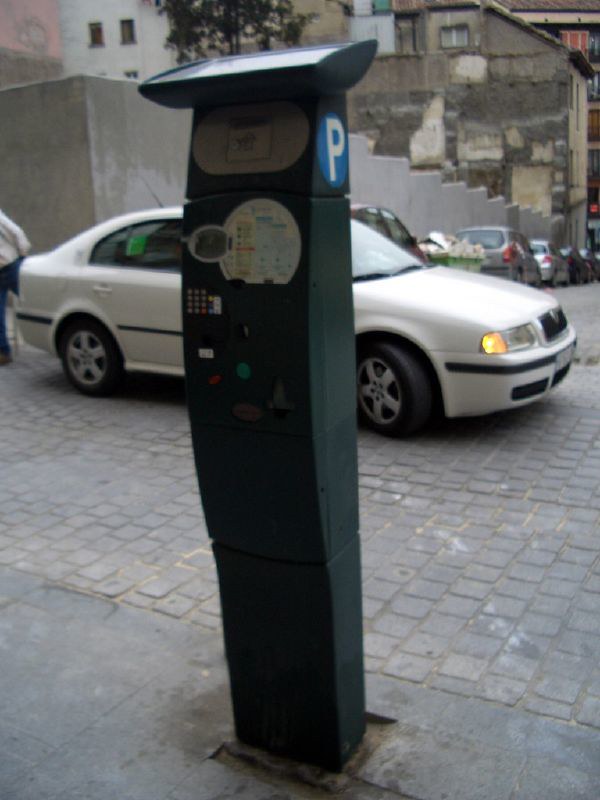The photograph captures an urban street scene, likely in a European city. The background is composed of a series of buildings, including an off-white one to the upper left and a dark gray one with patched cream-colored spots on the right. In front of these buildings runs a long, dark gray retaining wall that extends from the left edge towards the back right of the image. Lining the retaining wall are several cars parked facing away, in sequence: a black car, a yellowish garbage can, a gray car, another white car, and two black cars.

In the foreground, a smooth, light gray brick-paved road stretches across the image, bordered by a cement sidewalk. Driving along this road, heading towards the right, is a four-door white vehicle. Dominating the front foreground is a distinct greenish parking meter kiosk. This tall and rectangular meter has a blue circle with a white "P" on the top right, indicating its function. It features a keypad for entering payment information with nine buttons and a slot for card payments. Additionally, instructions on its operation are likely displayed on stickers at the top, complemented by a black solar panel crowning the unit.